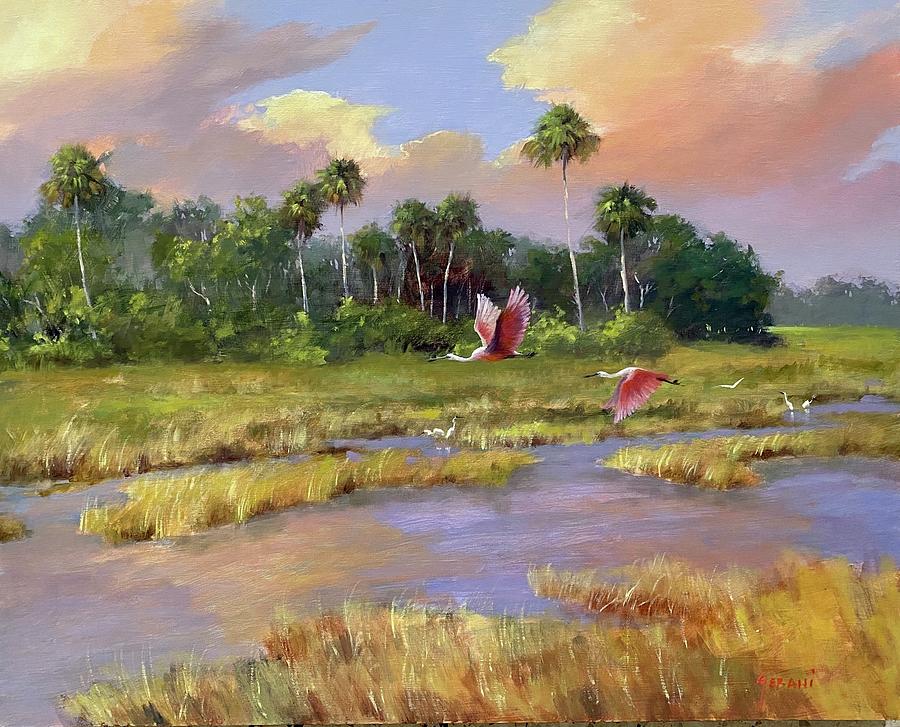This enchanting painting, depicting a serene wetland at either dawn or dusk, beautifully captures the ethereal interplay of light and nature. The sky, painted in a harmonious blend of warm pink, soft yellow, and serene blue hues, is reflected in calm waters dotted with lush green grasses and reeds. Central to the painting are two large birds, possibly herons or egrets, with striking white and pink feathers and black beaks, caught in majestic mid-flight with wings spread wide. These birds, alongside a few distant white ones either wading near the water's edge or elegantly flying low over the wetlands, add a dynamic element to the tranquil scene. Towering palm trees in the background enhance the tropical atmosphere, which some might even describe as prehistoric due to the painting's evocative style and vibrant color palette. The carefully rendered brush strokes bring texture and life to details, such as the feathers and leaves, while the bright blue sky interspersed with fluffy white and pink clouds suggests the delicate use of watercolor techniques. Additionally, a small, difficult-to-read red signature in the bottom right corner adds a personal touch from the artist, completing this clear and luminous portrayal of nature's beauty.